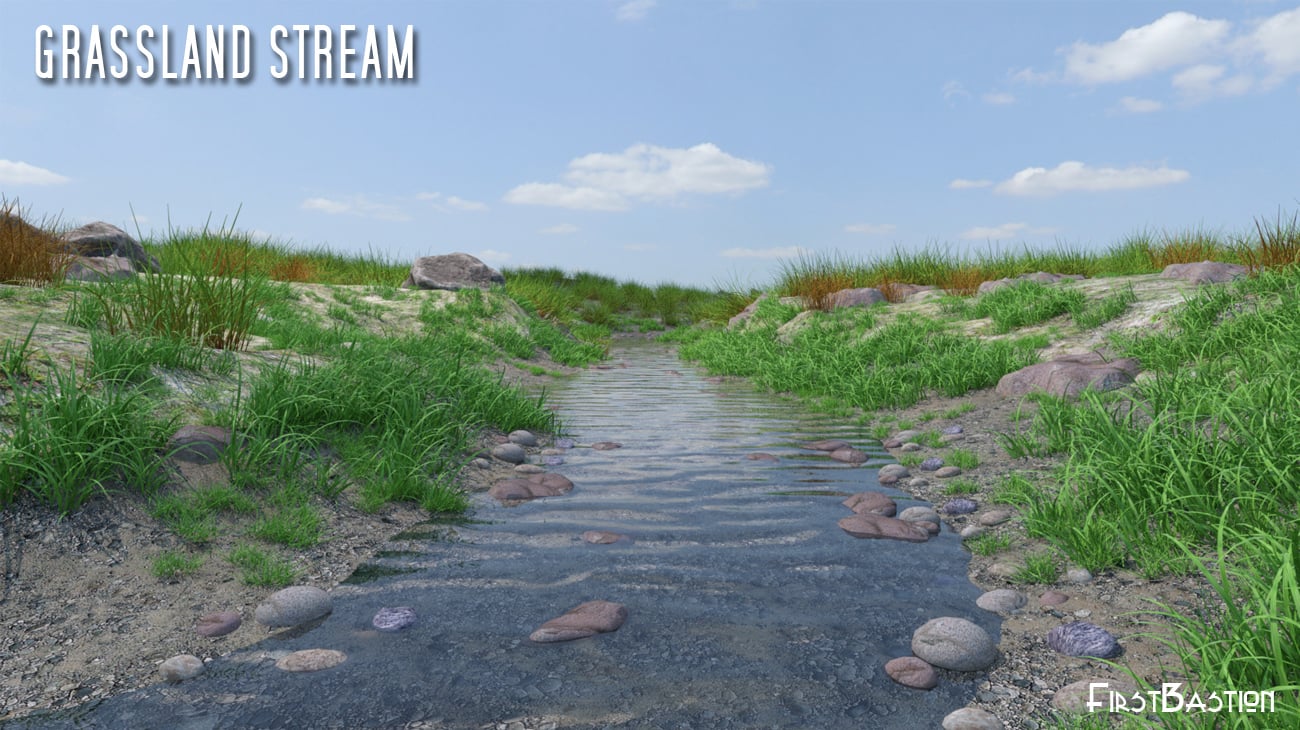This photograph captures a serene grassland stream scene on a clear, sunny day. In the upper left corner, white text identifies it as "Grassland Stream," while the lower right corner reads "First Bastion." The composition features a narrow stream running from the bottom edge to the mid-section of the image, flanked by tufts of crabgrass, patches of soil, and scattered rocks of varying gray and brown hues. The grassy banks rise gently on either side, suggesting a valley or hillside setting. Above, the sky dominates the top portion with its brilliant blue expanse accented by sparse, wispy clouds. The colors throughout the image include shades of blue, white, brown, and gray, contributing to a somewhat uncanny or digitally enhanced quality. Overall, the scene is simple and unassuming, with a focus on natural elements rather than dramatic or picturesque beauty.